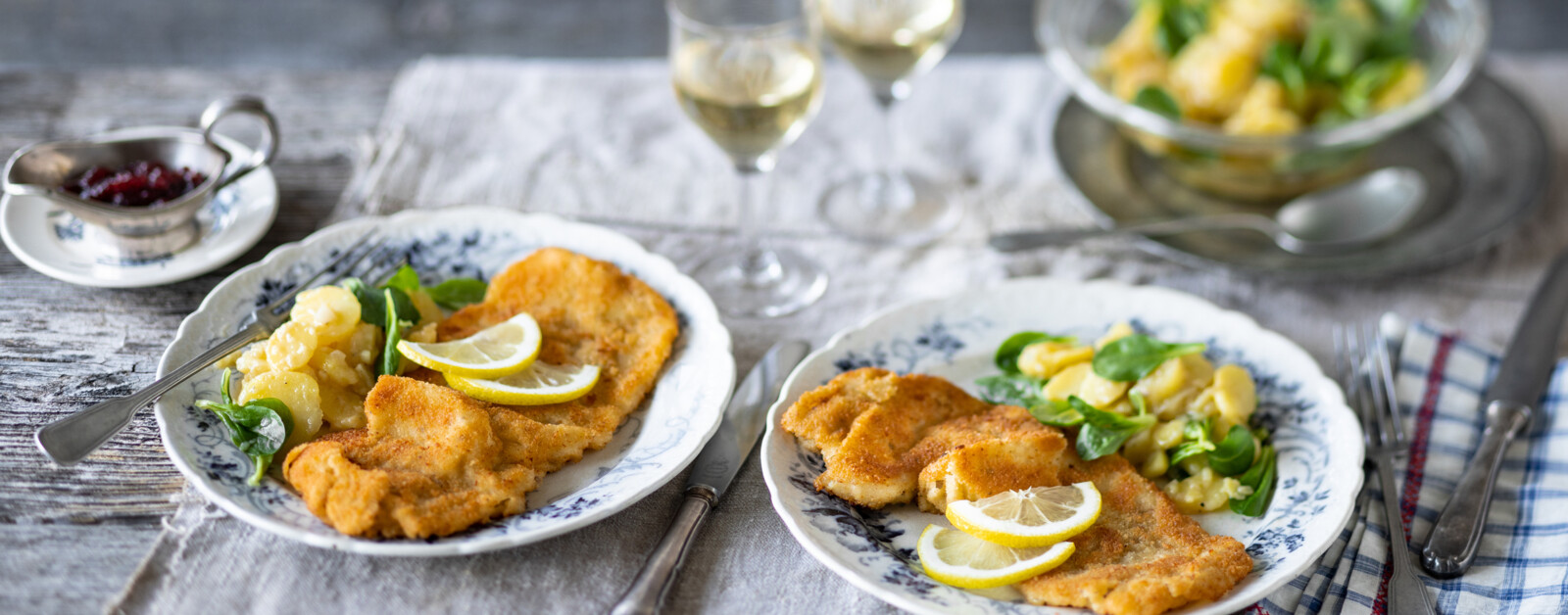This close-up image captures an elegantly arranged tablescape set on a rustic light wooden table. The focal point features two white plates adorned with a delicate blue floral design, each meticulously plated with thinly sliced, breaded fried fish topped with two thin slices of lemon. Accompanying the fish is a vibrant vegetable medley, adding a splash of color and freshness to the dish. The silverware is neatly placed on either side of the plates, resting on white napkins with a blue plaid design and a distinctive red line running down the side. In the background, the image subtly showcases blurred elements, including additional vegetables and two filled wine glasses, which appear clear and yellow. A small, gravy boat-like dish, possibly containing a berry topping or cranberries, adds an additional layer of culinary interest to the scene. This professional and appetizing presentation, with its crisp white and blue color scheme, exudes a refined and inviting ambiance, making it ideal for a cookbook or a recipe blog.